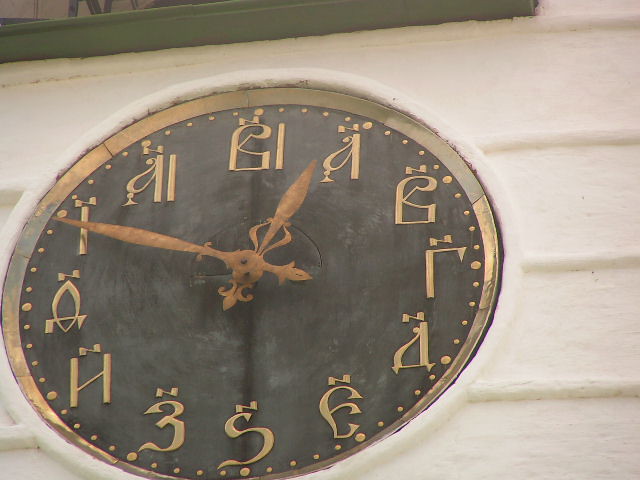Here we have a distinctive and unusual clock mounted on a textured white stone wall. The white background features a striped pattern with slightly raised ledges that encompass the clock. Just above the clock is a green ledge that juts out subtly, adding an interesting architectural element. The clock itself has a black face adorned with hands that are an intriguing shade of rust-like brown. It currently shows the time as 12:50. The clock's numbers are not in a conventional numeral system; instead, they are represented by unfamiliar golden symbols. The first symbol resembles an "A" with an accent above it, the second appears almost like a "P" with a curved line and a rectangle underneath, and the third looks somewhat like an "R." The precise origin of this alphabet is unclear, adding to the clock's enigmatic and exotic allure.